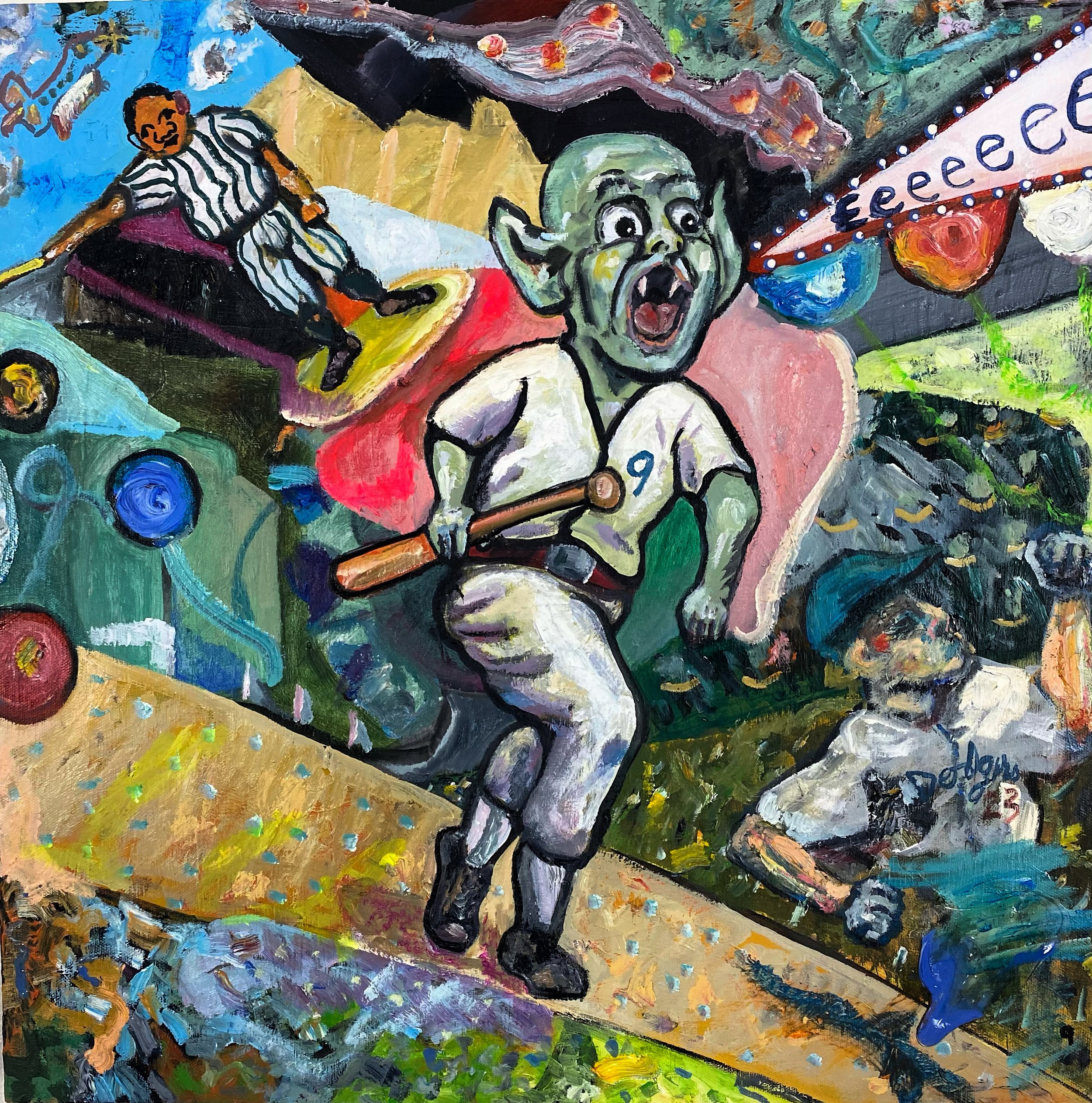This vibrant, abstract painting incorporates a lively mix of cartoonish and realistic elements, resulting in a dynamic depiction of a baseball scene. Dominating the center of the image is a green ogre, whose monstrous features include big ears and two sharp fangs exposed as he shouts the letter "E" repeatedly. Clad in a white baseball uniform marked with the number 9, the ogre wields a bat in an animated pose. To the left, an African American figure dressed as an umpire dons vertically striped attire, extending his arm authoritatively. On the right, a more traditionally human baseball player, highlighted by bright whites and vivid colors, is seen in motion wearing a Dodgers uniform with the number 22. The chaotic background features swirls of various colors, interspersed with lines, dots, and shapes like circles, evoking a child's exuberance yet executed with a sophisticated tone. Blue birds outlined in black flit around the top left, adding to the whimsical and eclectic feel of the artwork.